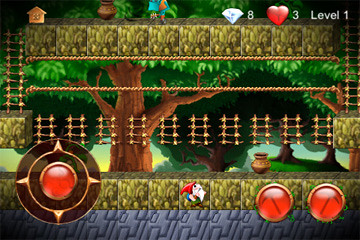The image is a detailed screenshot from an old 2D console game, prominently displaying pixelated graphics. The central character, resembling a gnome with a red pointy hat, white beard, or hair, stands at the bottom of the screen. Surrounding him are lush, large trees with big brown trunks and leafy green canopies, set against a bluish sky that peeks through the dense forest background. At the top left corner, there's a generic brown house, adding to the rustic atmosphere. The ground beneath the character is blocky, green grass, darker at the left and right corners.

The user interface elements are scattered across the screen. On the left side, there's a golden circular icon with interior arrows pointing up, down, left, and right, suggesting possible touch controls. Nearby are two red buttons, mirroring another pair of red circles on the bottom right, surrounded by golden lines. A tan pot is slightly above these buttons. The screen also features several small ladders and ropes extending across it, indicating possible pathways or obstacles.

In the upper right corner, the status bar displays crucial game information: the player has eight diamonds, denoted by a diamond icon with the number eight next to it, and three hearts symbolizing lives, right next to the "Level 1" label, all written in white font. The overall scene, with its cartoonish yet nostalgic appearance, vividly depicts a moment in a forest adventure game.